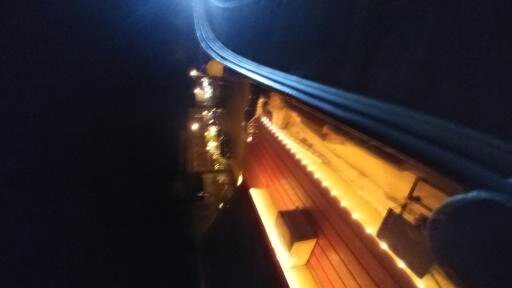This nighttime color photograph is quite blurry and two and a half to three times as tall as it is wide. The image is dark, dominated by deep shadows. It seems to capture the edge of a platform or possibly the bed of a vehicle, with a navy blue surface featuring a blue rim on its edge to the right. Adjacent to this edge are two long yellow objects that appear to be plastic and a gold, flower-shaped object attached to them. Next to these items is a dark blue circular object. 

In the lower portion of the image, there is a notable dark gray line starting from the center bottom, curving upwards towards the center right. This line transitions into a nearly rectangular, uneven yellow surface, potentially part of a building or another structure. Just to the left of this surface, there is a wooden plank adorned with tiny round lights, reminiscent of string lights but solid in color. This plank also supports a brown box-like shape. Further in the distance, towards the center of the image, faintly lit buildings are visible, contributing to a minimal glow against the otherwise dark backdrop.